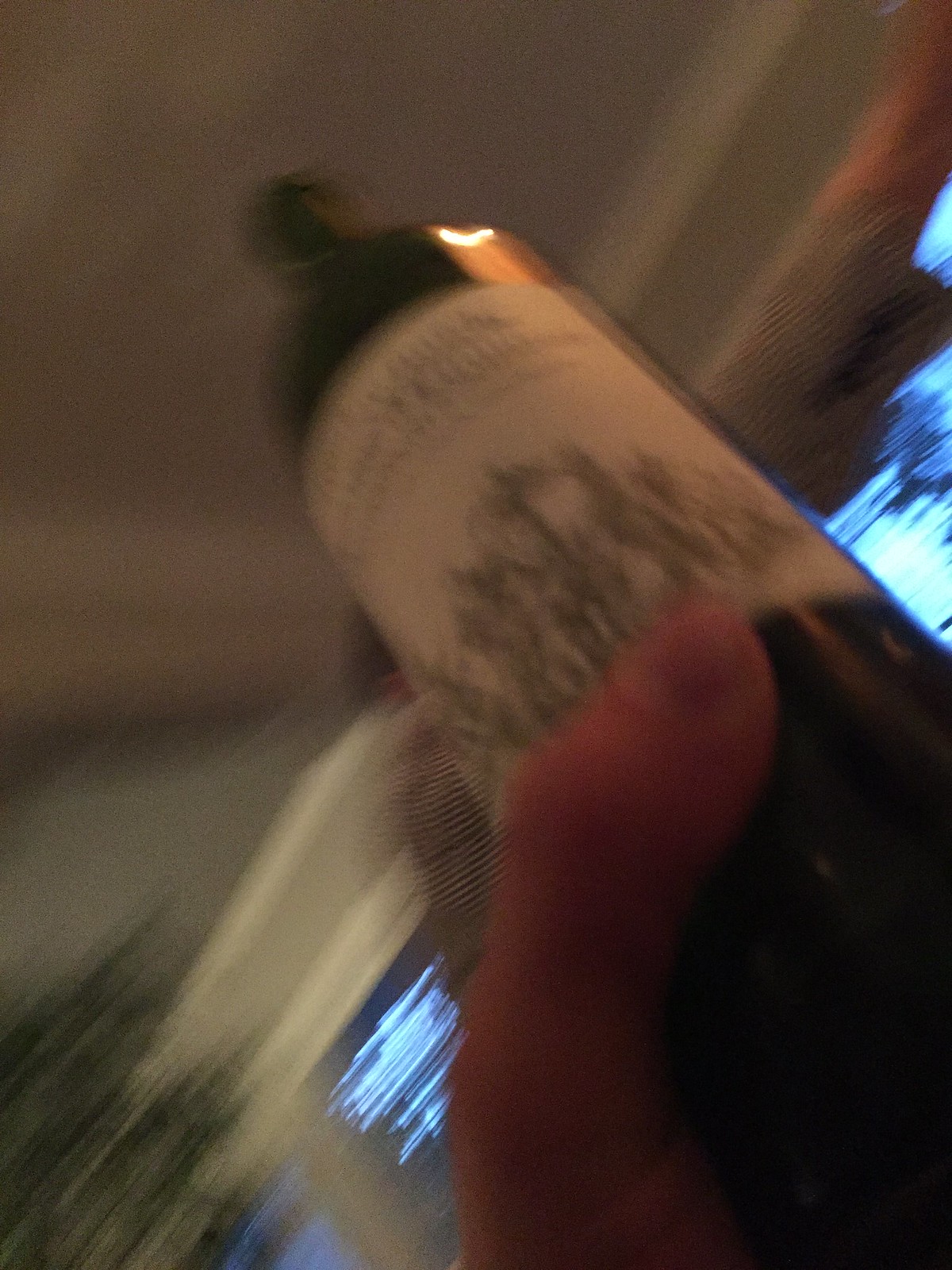The image captures an upward view of a dark-colored wine bottle, prominently positioned starting from the bottom right corner. The photo is notably blurry. A thumb, emerging from the bottom, grasps the bottle, showing the upper side along with the nail. The wine bottle features a white label in its center, which is blurred but reveals some tree-like designs at the bottom and text at the top. The bottle itself is encased in black glass, continuing to the top with a consistent black hue. Additionally, a faded green plant appears in the bottom left corner. In the background, there are a couple of windows emitting blue light, situated between the wine bottle and the ceiling, which is painted in a plain gray color.